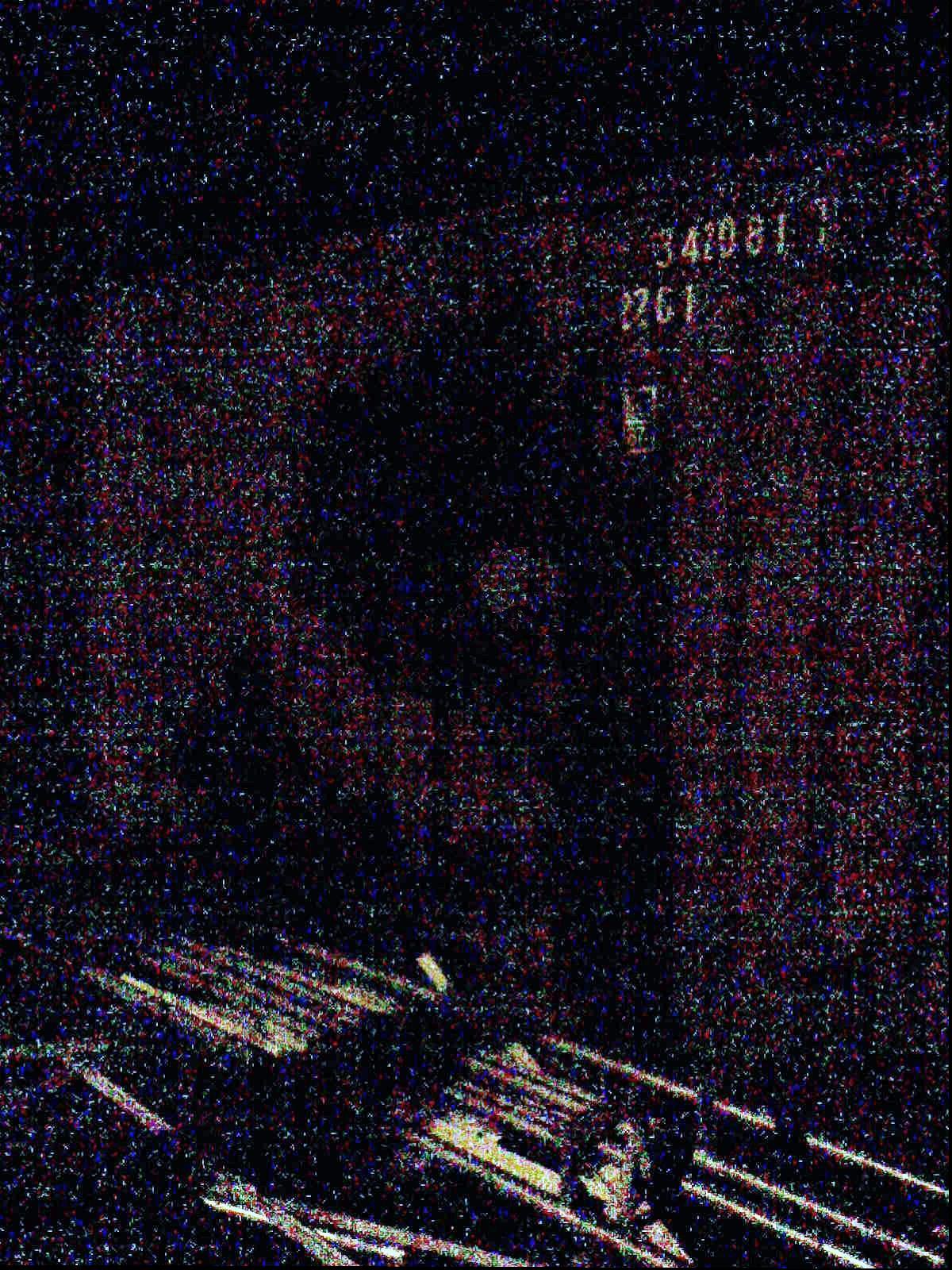The image, captured in portrait mode, is characterized by extremely dark tones and a high level of pixelation, obscuring distinct details. The backdrop is pitch black, and the frame is scattered with numerous brightly colored dots. These dots are densely packed within the central two-thirds of the image, becoming more sparsely distributed as they ascend towards the top. At the bottom right corner, several pixelated light-colored lines slant slightly upwards towards the left. Additionally, near the top right corner, two sequences of numbers are visible, reading "341081" and possibly "2261".